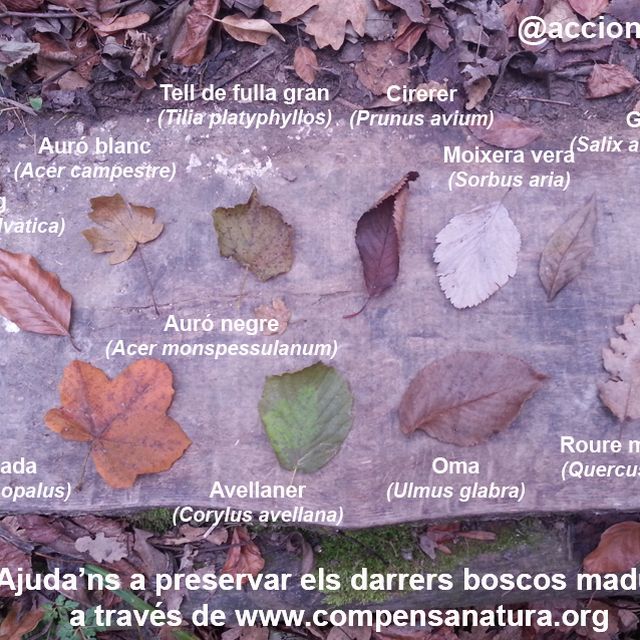The image presents an array of variously colored leaves meticulously arranged on a piece of stone. Each leaf is labeled with both its common name and scientific name, showcasing botanical diversity. From left to right and top to bottom, the labels include 'Auro Blanc' and 'Acer Campestre', followed by 'Tel de Fula Gran' or 'Tilia Platyphilos'. Notably, 'Prunus Avium', labeled in Spanish as 'Cirer', appears prominently. Another leaf labeled 'Moxiera Vera' or 'Sorbus Aria' is distinctively white. Additional labels seen are 'Oma' or 'Ulmus Glabra' and 'Avelanere' or 'Corylus Avellana', with some labels partially obscured. A message in white text at the bottom of the image reads "Ayudas a Preservar el Darreres Boscos Madre a través de www.compensanatura.org". The scene is set outdoors, with fallen leaves on either side of the stone suggesting a natural setting.